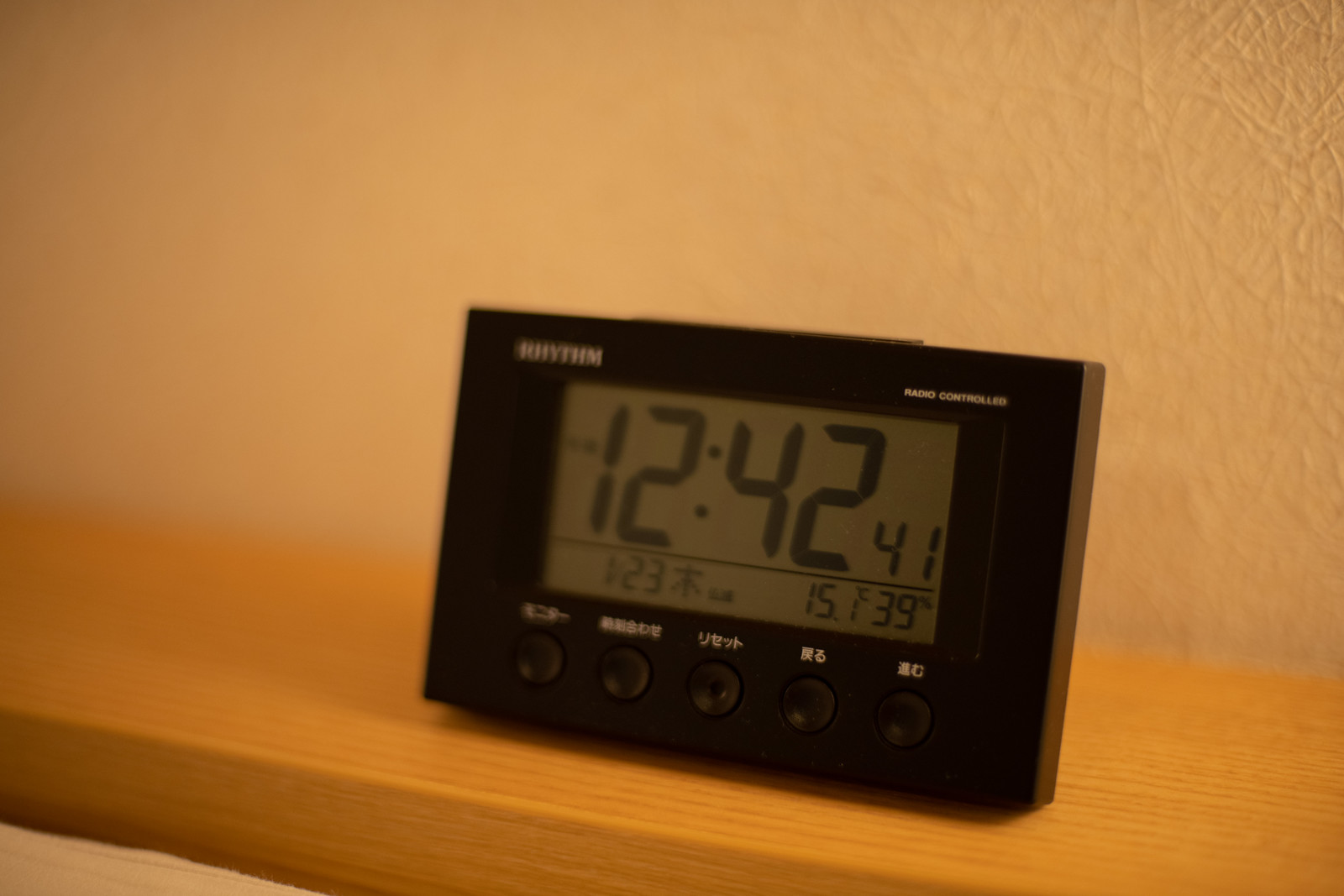In this sepia-toned photograph of a bedroom, a new-looking light brown wooden headboard spans the lower part of the image from left to right. Atop the headboard, centrally located but slightly shifted to the right, stands a sleek, black digital alarm clock. The clock features a vertical, slim design with a black border and white lettering; though the brand name in the top left corner is indiscernible. The digital display shows the time 12:42:41 in black digits against a grey background, with additional numbers, possibly representing a calendar or temperature, aligned below it. The wall behind the headboard is painted white and covers the upper background of the image. A small portion of a white mattress is visible in the bottom left corner, contributing to the cozy bedroom setting.